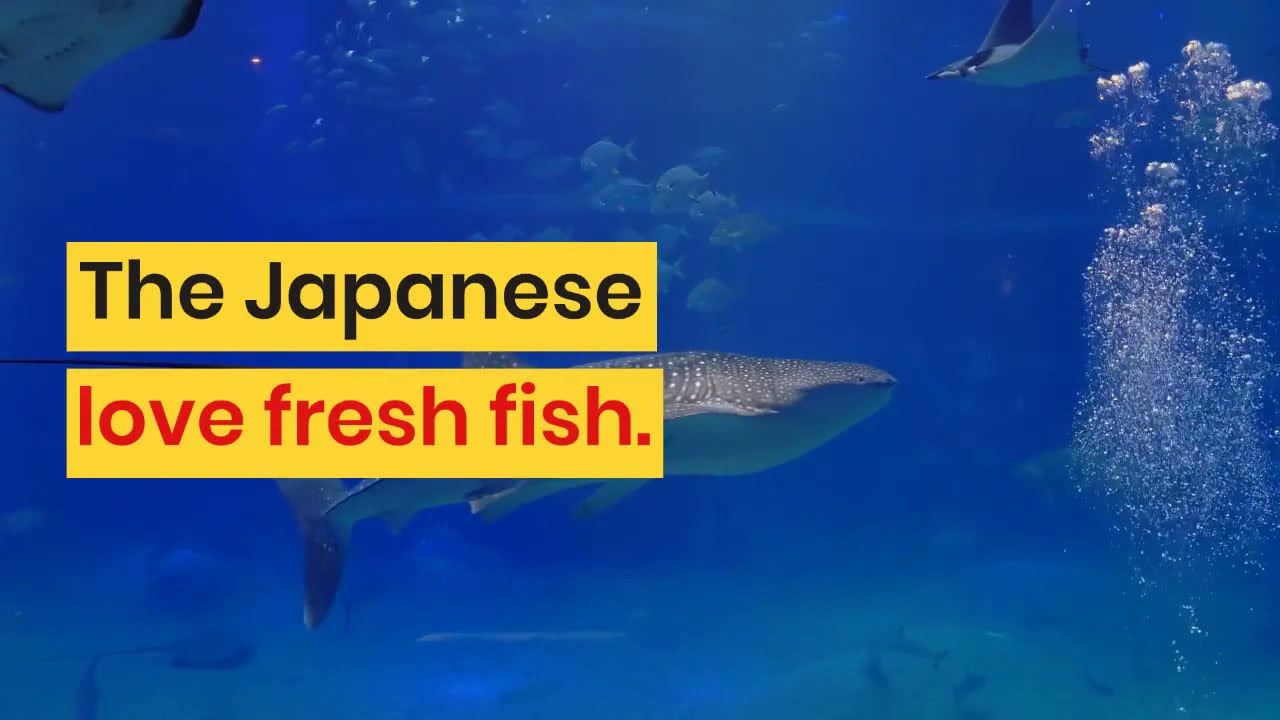In this underwater scene, the image predominantly features a vast expanse of blue ocean. At the center, a large gray fish, speckled with white spots, swims towards the right. Above it, a school of smaller fish is visible, heading in the opposite direction. The upper right corner showcases a manta ray gliding to the left, while the top left corner reveals the underside of another manta ray. The bottom of the scene resembles a sandy ocean floor with wavy sand formations. On the right side of the image, a stream of bubbles rises through the water, possibly from a scuba diver below. Two yellow rectangles on the left side contain Japanese text in black, and underneath, in another rectangle, the red text reads "love fresh fish."